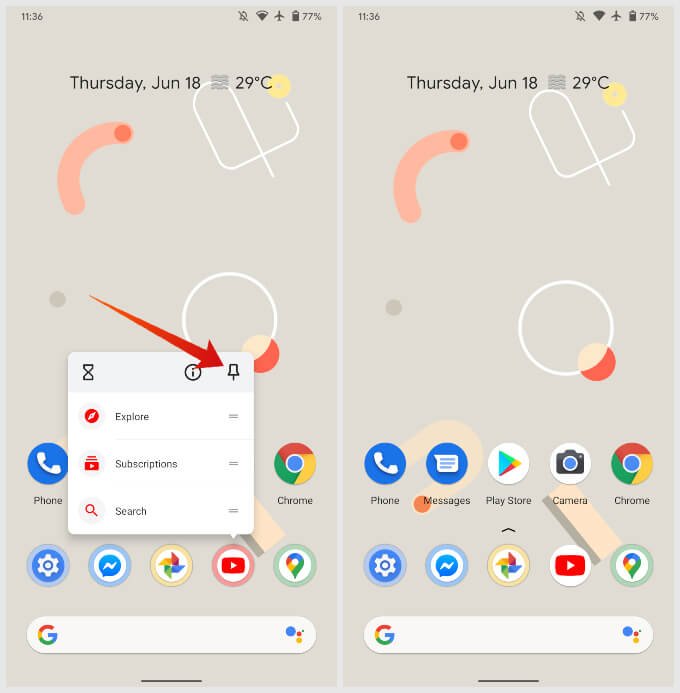This image is a side-by-side screenshot of a mobile phone, shown from two different angles. Both angles display the same beige background and abstract wallpaper featuring pink circles and a semicircle. The phone's status bar shows the time as 11:36 AM on the top left, with a battery level of 77% on the top right. Below the time is the day and date, "Thursday, June 18," and a temperature reading of "29°C."

In both screenshots, several app icons are visible, including Google Chrome, Phone, Google Photos, YouTube, and Facebook Messenger. At the bottom of the screen, there is a Google search bar.

The image on the left differs, featuring a pop-up window with options labeled "Explore," "Subscriptions," and "Search." A prominent red arrow points to a pin icon located at the top right corner of this pop-up window. The detailed layout and visual cues in the screenshots provide a clear and comprehensive view of the phone's interface and functionalities at that moment.